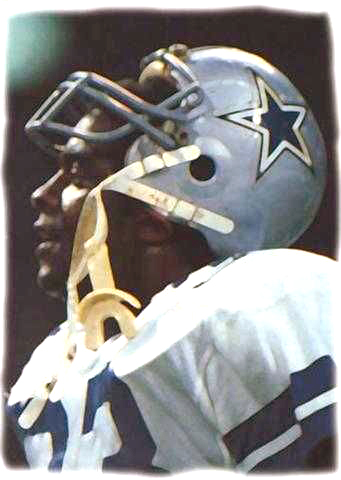The image is a small, vertical, rectangular close-up of a black male football player. He is wearing a white sports jersey with a blue letter and possibly the tops of the numbers '2' or '8', though the full numbers are not visible. The jersey has blue stripes on the sleeves. His silver-colored helmet, featuring a blue star with a white and another dark-colored border, is lifted up, revealing his face. The background of the photo is blurred and indistinct, providing no additional context. The photo frames the player from the chest to just above the helmet, focusing solely on the upper part of his body.